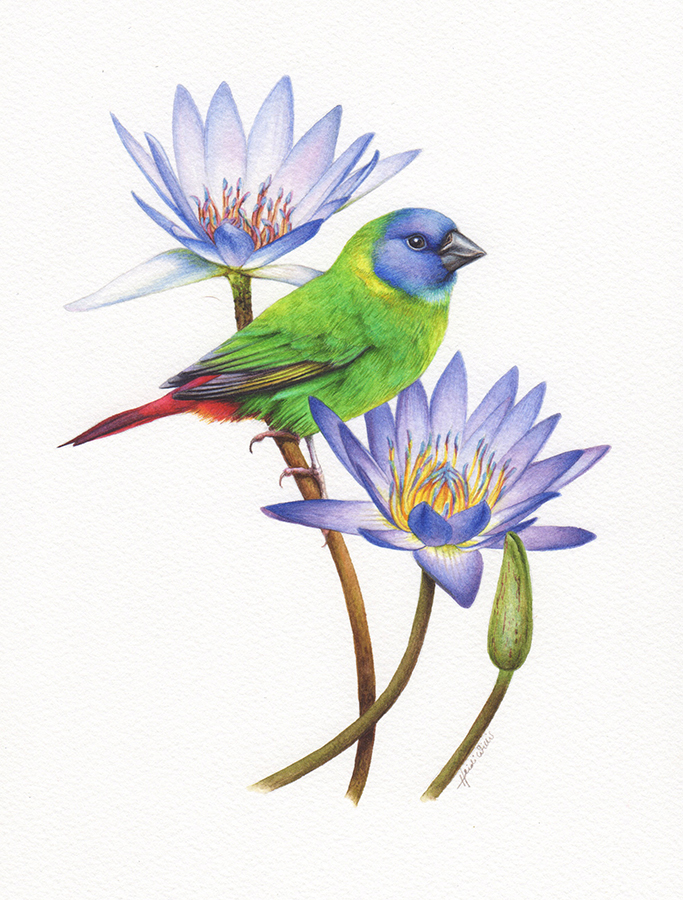This artwork, rendered on a textured white canvas, features a meticulously detailed bird perched centrally on a stem with vibrant flowers. The bird, likely a wren, is depicted with a green body and a distinctive blue face, complemented by black eyes and a charcoal black beak. Its tail feathers are vividly red, with accents of pink, black, and some yellowish hues that add depth to its form. The bird’s talons, darker in color, grasp the stem securely, which also supports two main blossoms and an unopened bud.

The foremost flowers, both displaying thin, teardrop-shaped petals, exhibit a stunning blend of purple and light blue shades, with reddish-yellow pollen visible within the blossoms. The stems supporting the flowers and the bird are a mixture of green and brown, adding a naturalistic touch to the scene. The arrangement places one flower above and another below the perched bird, creating a balanced composition.

Interestingly, a smaller, unopened bud with a green stem is positioned adjacent to the developed flowers. The artist, identified by the signature "Heidi Willis" at the bottom right corner of the canvas, has skillfully blended pencil, pen, or potentially watercolor techniques to create this lifelike and colorful portrayal of the bird amid its floral environs. The background remains a clean beige-white, enhancing the delicate colors and intricate details of the main subjects.